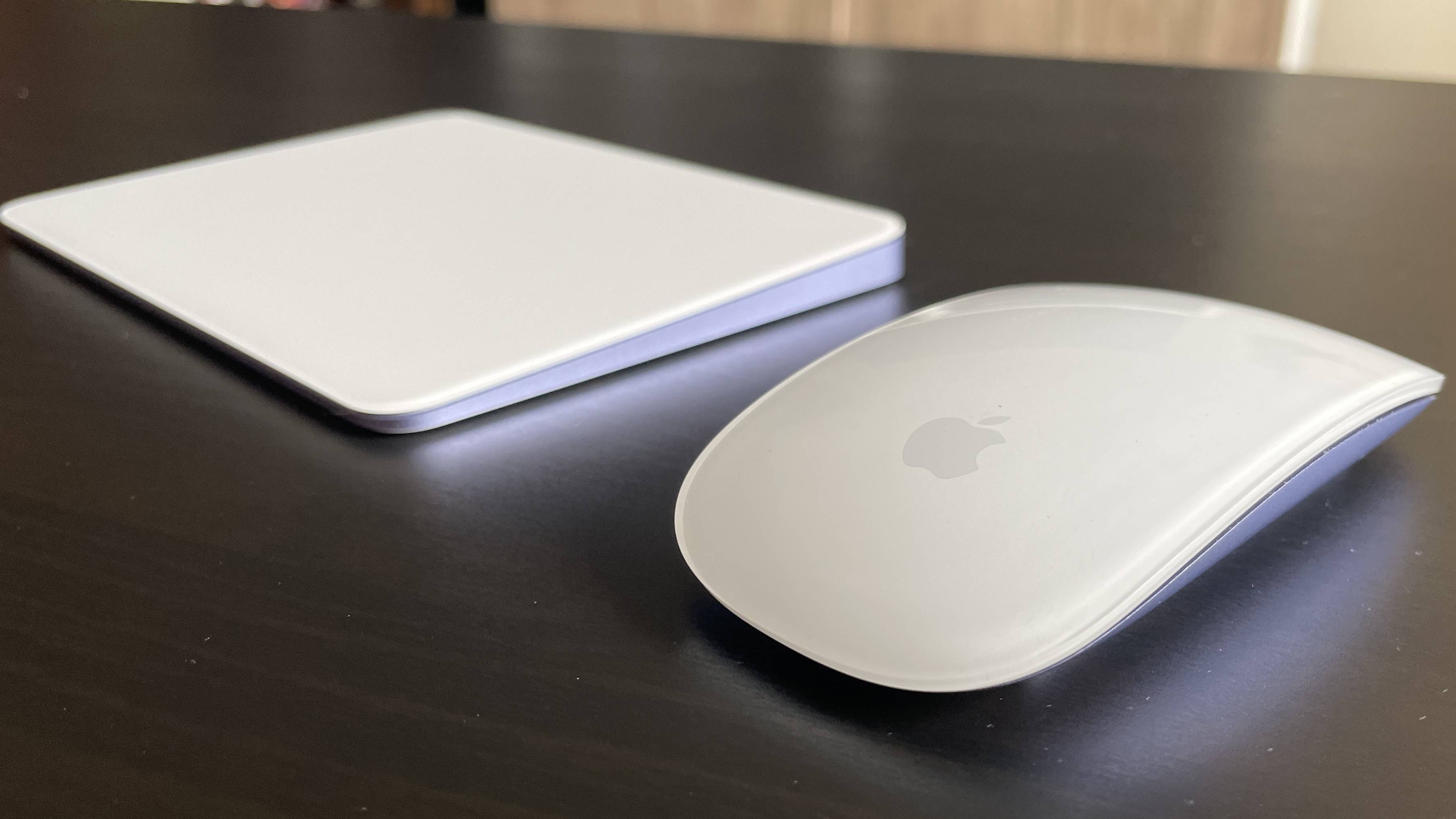This detailed photograph captures a minimalist setup on a dark brown wooden desk that is impeccably clean. The focal point lies in two sleek Apple products centered prominently in the shot. On the right, there's a pristine white Apple mouse, distinguished by its curved, glossy surface and the iconic Apple logo. This mouse, devoid of traditional buttons or scroll wheels, exudes a modern, streamlined design, tailored for smooth navigation. Beside it, to the left, is a flat, rectangular white object roughly the size of a small notebook or closed laptop. There is some ambiguity regarding this item's exact function: it lacks an Apple logo, leading to guesses ranging from a touch-sensitive keyboard to a charging pad, without visible buttons or screens. The composition features a dark wooden backdrop, suggesting the setting might be an office or a workspace, providing a stark contrast that highlights the sophisticated simplicity of the Apple devices.